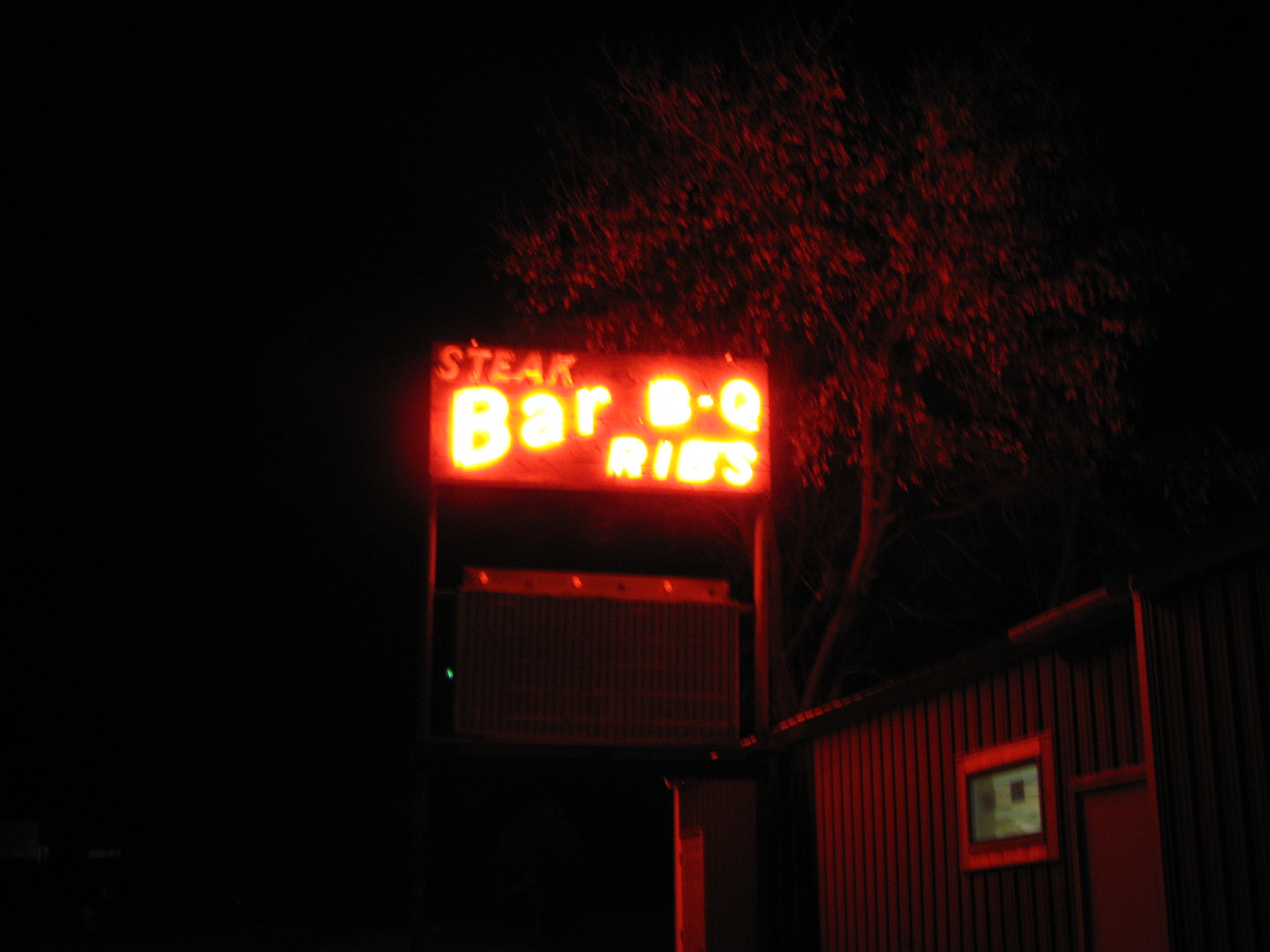A photograph captures the exterior of a building, possibly a business, at night. Dominating the scene is a sign with two lines of text: "steak" and "barbecue ribs," written in fluorescent orange letters. Notably, only the phrase "barbecue ribs" is illuminated, casting a warm reddish glow against the darkness. This light subtly bathes a nearby tree and the side of the building with a soft, reddish hue. The building itself features a small rectangular window adjacent to the entrance, standing out amidst the otherwise dark surroundings. The overall ambiance of the image is characterized by the stark contrast between the vivid sign and the enveloping night.